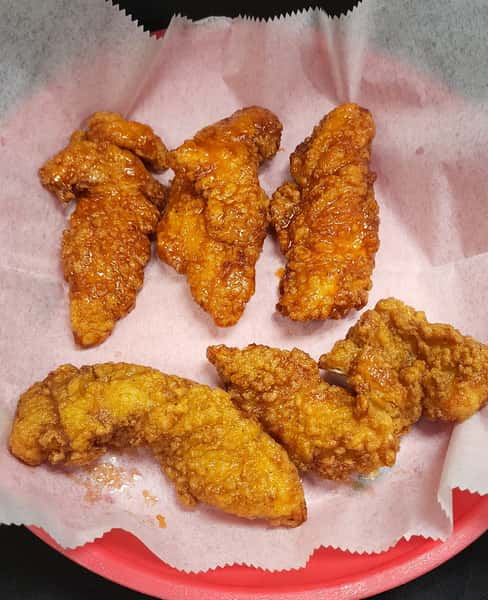This color photograph features a vertically oriented rectangular image centering on a collection of fried foods. The background is a deep black, creating a stark contrast that highlights the vibrant colors of the dish. The food is presented on a pink plate, which closely resembles an oval shape. Lining the plate is a crumpled and separated piece of white paper, presumably used to absorb excess grease. 

On top of this paper, there are six pieces of food, which appear to be breaded and deep-fried chicken tenders. The arrangement is somewhat structured, with three vertical pieces positioned in a row at the top, and two horizontal pieces at the bottom, slightly overlapping in the middle. The tenders showcase a range of golden brown hues with a slight sheen, indicating their crispy fried texture.

The image distinctly lacks any accompanying bowls or dipping sauces, focusing solely on the fried chicken tenders. The entire composition is centered within the frame, and the red plate occupies the majority of the image, suggesting either a kitchen or restaurant setting. The absence of other elements directs all attention to the texture and golden coloration of the fried chicken, making it an appetizing and visually appealing presentation.